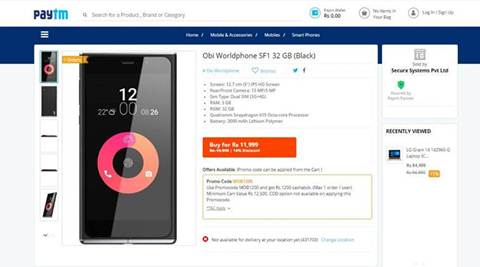At the top of the image, there is a header that appears to say "Pay FM" or "Pay TM," though the text is somewhat unclear. To the right of the header, there is a search box followed by three elements that are too blurry to identify. Below this, there is a dark blue navigation bar that clearly displays the word "Home," while the remainder of the text is too blurry to decipher.

Below the navigation bar, the text reads "OB World Phone SF1 32GB Black." Underneath this line, there is a heart icon. Accompanying this are several bullet points with descriptive text next to them. Beneath these details, there is an orange rectangle with more text inside, though the specific wording is not legible.

Further down, there is another box with text both above and within it. Below this section, a sentence is visible, but its content is not specified. To the left of this text, there is an image of a smartphone displaying the time as 12:00 and featuring a pink-colored circle on its screen.

Additionally, there is a photo gallery on the left side of the overall layout, showcasing smaller images of the same smartphone. On the right side, there is a section labeled "Previously viewed," which includes an icon and some accompanying text.